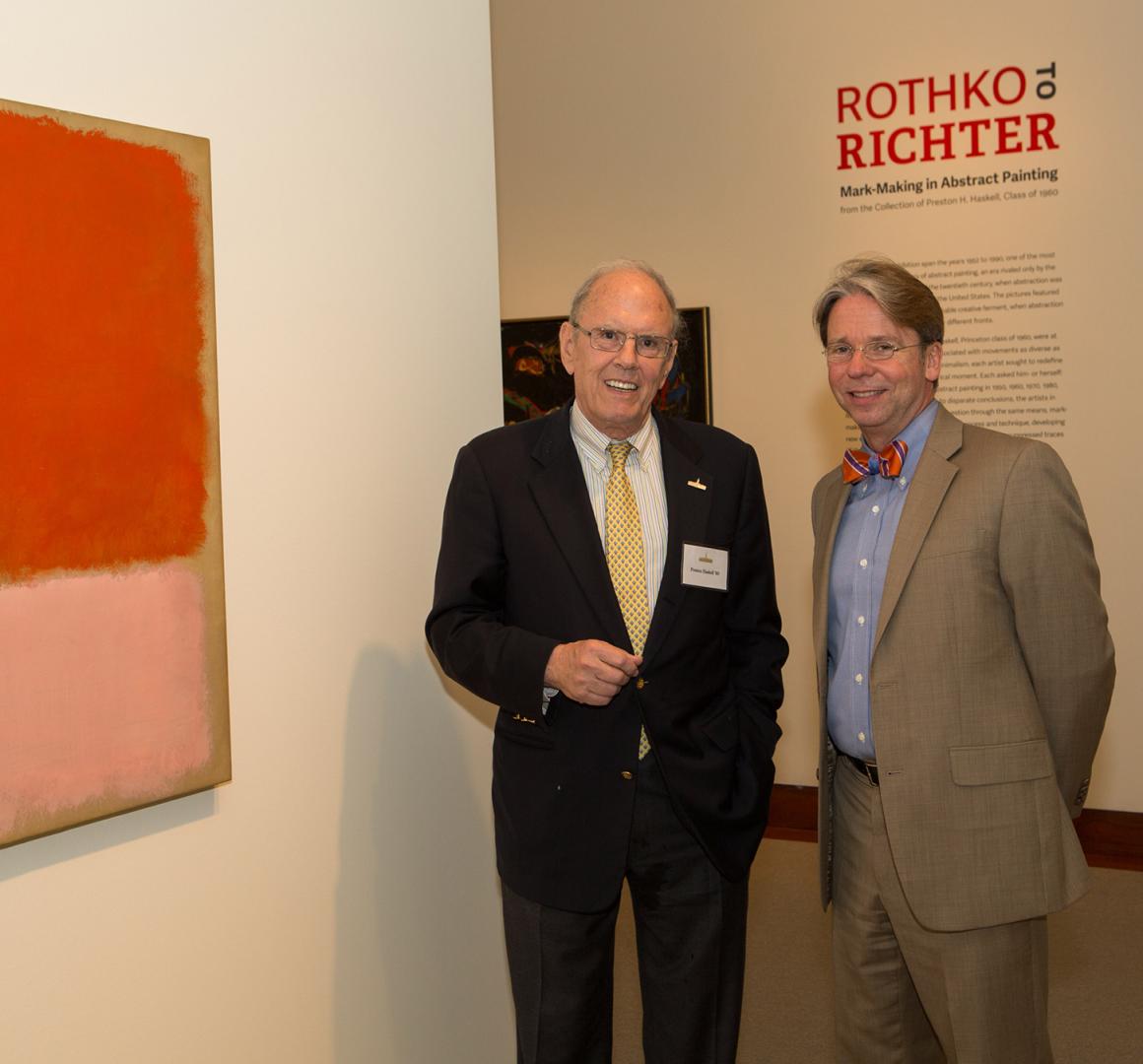In this image, two older gentlemen are posing together, likely at an art seminar or exhibit. The man on the left is dressed in a black suit with a white shirt and a yellow tie featuring a pattern. He is mostly bald with some gray hair, wears glasses, and is smiling. The man on the right is wearing a gray suit paired with a light blue button-up shirt and a red bow tie with blue and purple stripes. He also has grayish hair, glasses, and is smiling while holding his arms behind his back, giving off an academic vibe. 

Behind them, the exhibition wall features the text "Rothko to Richter" in red, followed by "Mark making in abstract painting" in black. The left wall showcases a painting by Rothko, marked by its distinctive color blocks - the bottom third in pink and the upper third in red. This detailed setting indicates that they are part of an exhibit focused on abstract painting techniques from notable artists like Rothko.